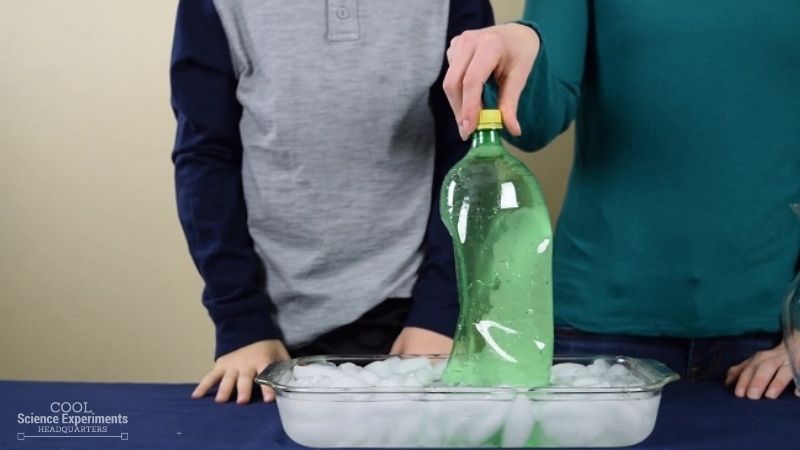In this detailed image, two individuals, visible only from the chest down, are engaged in a science experiment. The person on the left appears to be a younger boy dressed in a gray torso sweater with blue long sleeves, while the individual on the right, possibly a slightly older woman, is wearing a turquoise, bluish-green long-sleeved sweater. They both stand behind a blue felt-covered table, which holds a glass cooking tray filled with ice. The older person on the right is holding a green 2-liter soda bottle with a yellow cap, seemingly in the process of twisting off the cap. The bottle appears to be compressed, indicating a possible reaction or process involving the ice. The background features a plain beige wall, and in the bottom left corner, there's a watermark in white text that reads "Cool Science Experiment Headquarters."